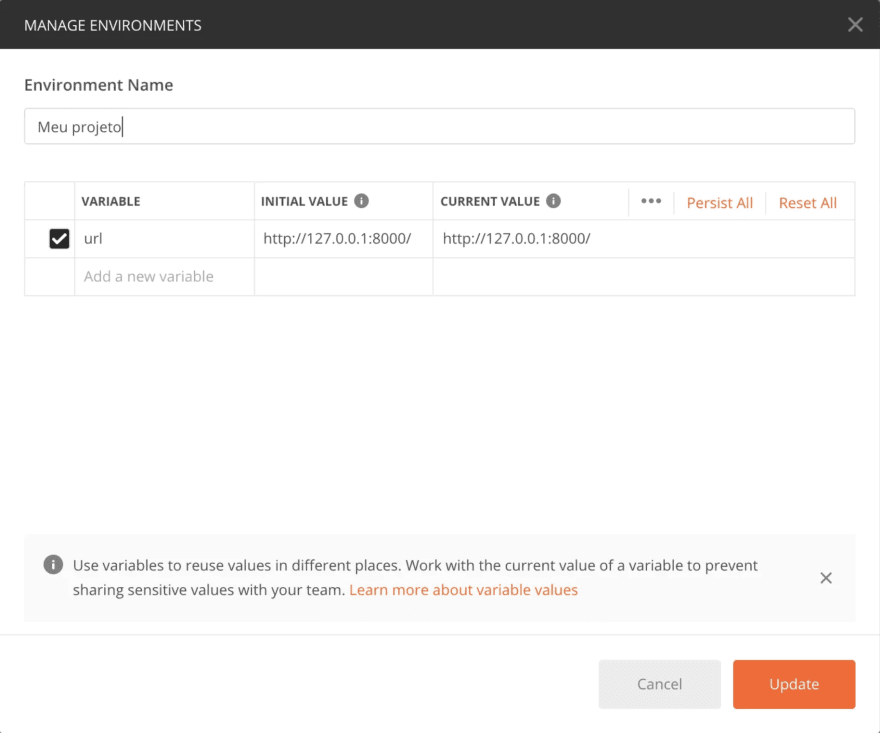The image depicts a webpage dedicated to managing environments within a software application. At the top of the page is a sleek black banner with the text "MANAGE ENVIRONMENTS" in bold, white, capital letters positioned on the left. To the far right of the banner is an 'X' icon, presumably for closing the page or section.

Below the banner, the background transitions to white. Prominently, the text "Environment Name" (or possibly "Environmental Name") is displayed, accompanied by a text box for inputting the name of the environment. Adjacent to this text box, the term "Menu" is displayed, followed by the string "P-R-J-E-T-O". A mouse cursor is visible nearby, indicating possible interaction.

Further down, the webpage features a data table or graph with several rows and columns. Each cell in the table is represented as a small square. Specifically, in the second row of this table, there is a square containing a white checkmark. The first row column headers are labeled "Variable" in bold text, followed by "URL". There is an option to "Add a new website" located in the third row. The columns also display "Initial Value" and "Current Value of the website", giving users the ability to compare and input data.

To the right of the table are three vertical dots (an ellipsis icon) suggesting a dropdown menu, and beneath it, options for "Persist All" and "Reset All" are highlighted in orange text.

Towards the bottom of the page is a light-colored banner featuring an information icon (a circle with an 'i' inside). This banner contains informative text: "Use Variables to Resort Values in Different Places. Work with the current value of a variable to present sharing sensitive values with your team." Additionally, there are links to "Learn more about variable values" emphasized in orange text. At the very bottom, two action buttons labeled "Cancel" and "Update" are available for user interaction.